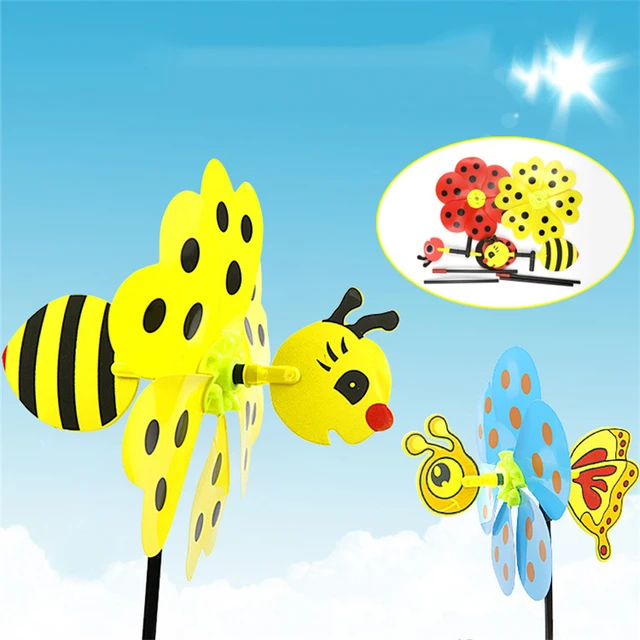This image is a detailed advertisement for whimsical yard decorations designed as a wasp and a butterfly. Both figures are constructed as windmill-like items, likely intended to spin when placed in the garden. The background showcases a vibrant blue sky with a white, star-shaped area representing the sun in the upper right corner, while a cloud-like white area blankets the bottom of the image. 

On the left side of the picture stands a wasp decoration. This playful figure is predominantly yellow, with black spots adorning its petal-like wind-catcher wings. It features a head with a yellow base, black antlers, and a red, cartoonish nose. The rear part of the wasp is striped in yellow and black. The wasp is mounted on a black stick designed to be inserted into the ground.

To the right is a colorful butterfly decoration. Its composition includes blue wings with red spots, further backed by additional red and yellow wings. The butterfly's head is yellow, complemented by yellow antlers, and it too has a similar stick attachment at the base for securing in the garden.

In the upper right corner of the image, there is an elliptical inset displaying two variations of the wasp. One is yellow with black spots, and the other is red with black spots. The inset also reveals an assembly process, showing the windmill components detached to expose the plastic stakes necessary for assembly and ground placement.

Together, these vibrant and functional decorations serve to add a playful touch to any outdoor space, capturing the viewer's attention with their bright colors and dynamic design.